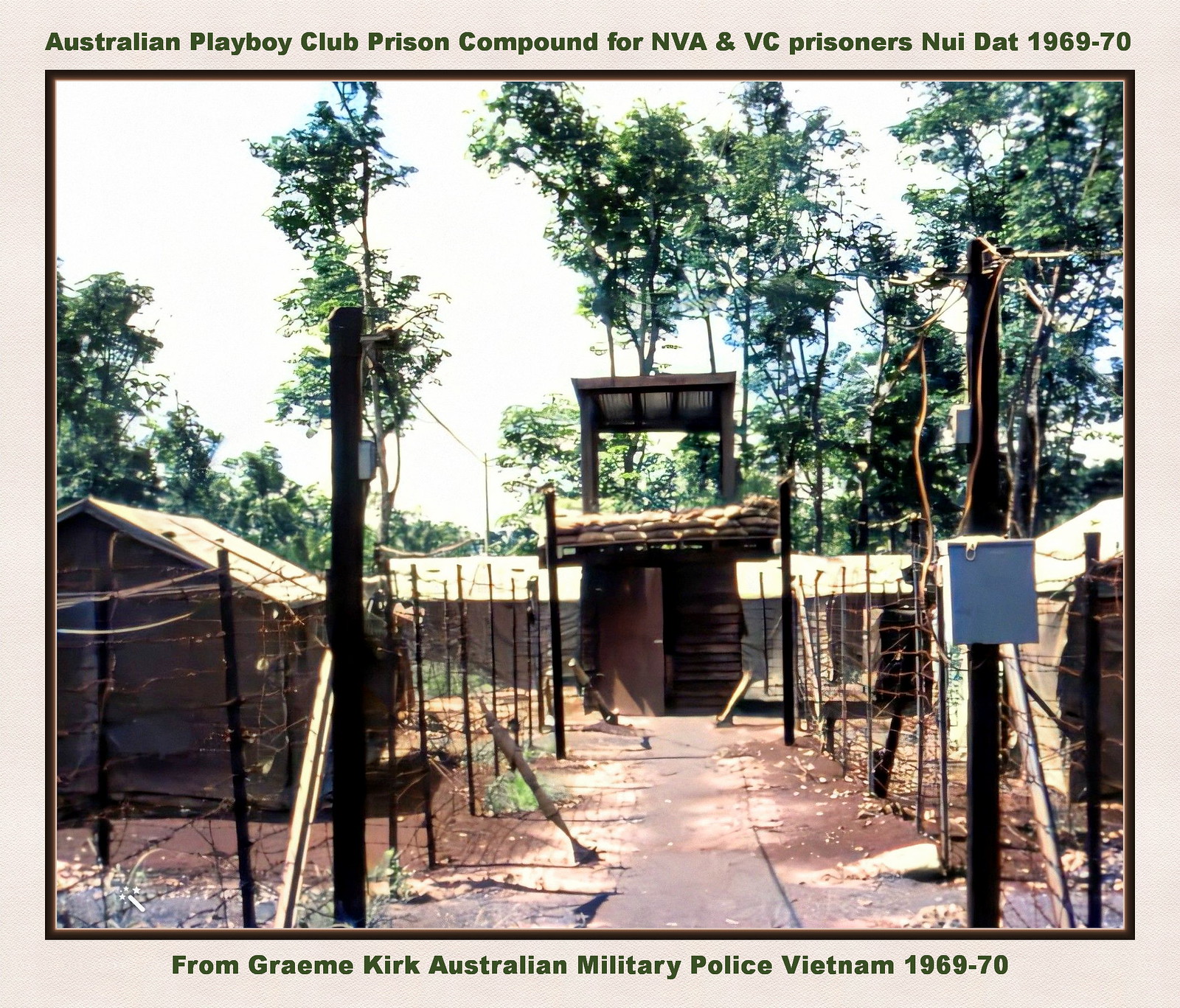The photograph, presented on a white background with a black frame, is captioned "Australian Playboy Club Prison Compound for NVA & VC Prisoners, Nui Dat, 1969-70" in green bold text at the top. Below the image, another caption reads, "From Graham Kirk, Australian Military Police, Vietnam, 1969-70." The photograph itself depicts a military prison compound located in a jungle or tropical setting. The foreground features a paved walkway leading to a two-story gatehouse with an open canopy above the first story. Surrounding the walkway are fences and barbed wire. In the background, there are low, one-story barracks and a large watchtower is centered within the compound. Trees and a nondescript sky form the backdrop of the scene. On the left side of the compound sits a cabin, while a tent is visible on the right.